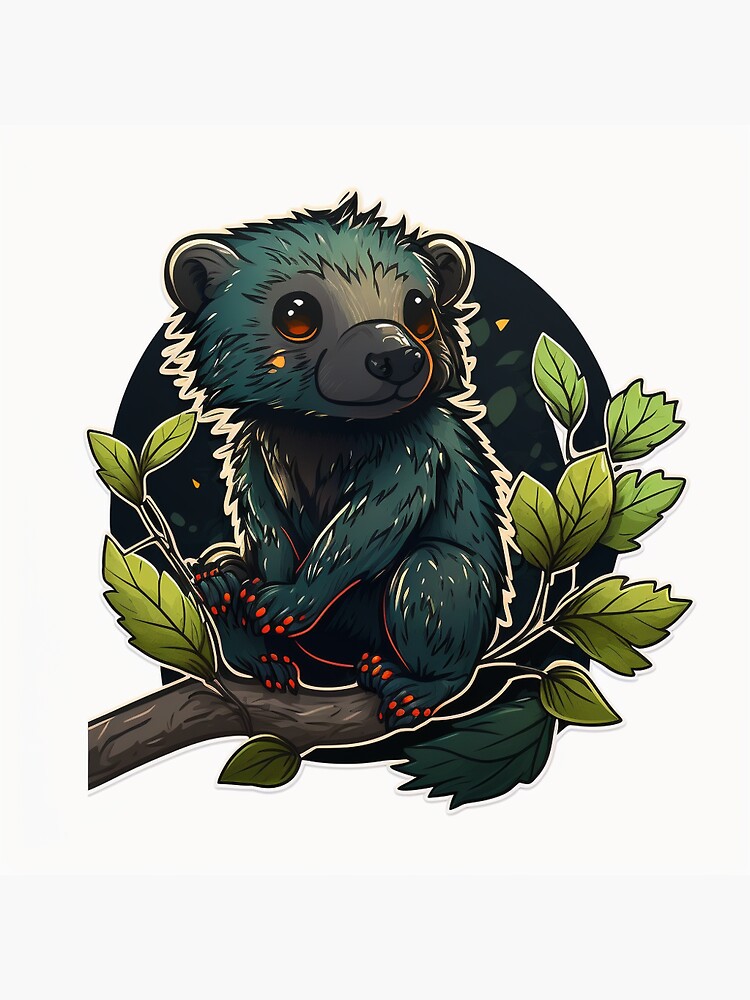This image features a vividly detailed painting of a bear cub perched on a tree branch. The cub's body, oriented towards the left, contrasts with its head turned back to the right, gazing intently with its reflective black eyes with white highlights. Its fur features a complex array of colors; predominantly light blue on the head and body, interspersed with speckles of white and patterned with black lines to depict fur texture. A distinctive light gray coloring adorns the area between its eyes and the inside of its perky ears, with the forehead echoing the light blue hue. Its muzzle is predominantly brown with light reflections and culminates in a black-tipped nose. The bear's claws, curiously painted orange, hover above the tree branch it sits upon, which is a rich brown extending from the left side of the painting. Surrounding the branch are vibrant light green leaves, framing the bear to the left and right. In the background, a dark black circle partially obscured by the bear contrasts with the overall off-white, very light gray background, creating a striking focal point. The entire composition is vertically rectangular, potentially indicative of a sticker or decal design.